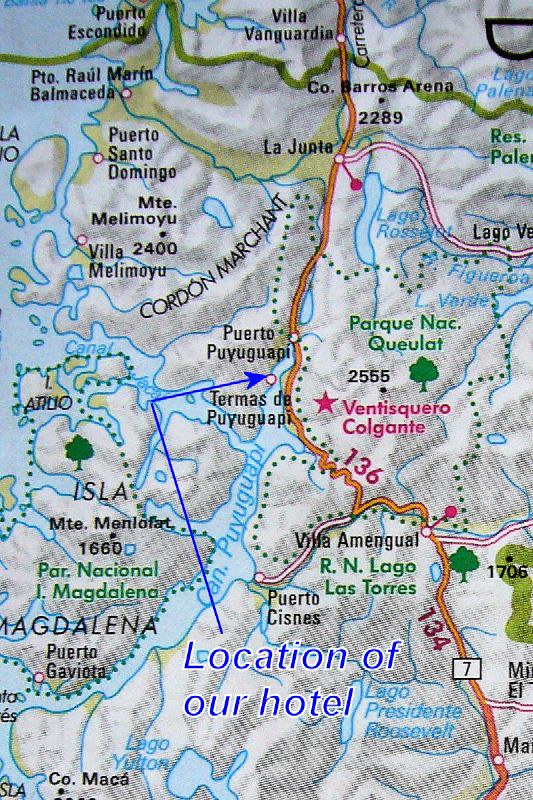The image is a detailed map in portrait orientation, featuring a significant amount of colorful labeling. The map uses various colors, including black, green, blue, pink, and orange, to highlight different features. A prominent blue arrow spans from the center left to the top center of the map, making a sharp right turn to point at a red dot, which is labeled "Termas de Puyugua pi." The label at the bottom of this arrow indicates "location of our hotel," emphasizing its importance. The map showcases both land and water, with rivers clearly depicted. The cities have Spanish names, suggesting the map might be of a location in a Spanish-speaking region such as Mexico, Spain, or Central America. The style of the map appears distinct from common American maps, possibly indicating the use of technology from a different country.